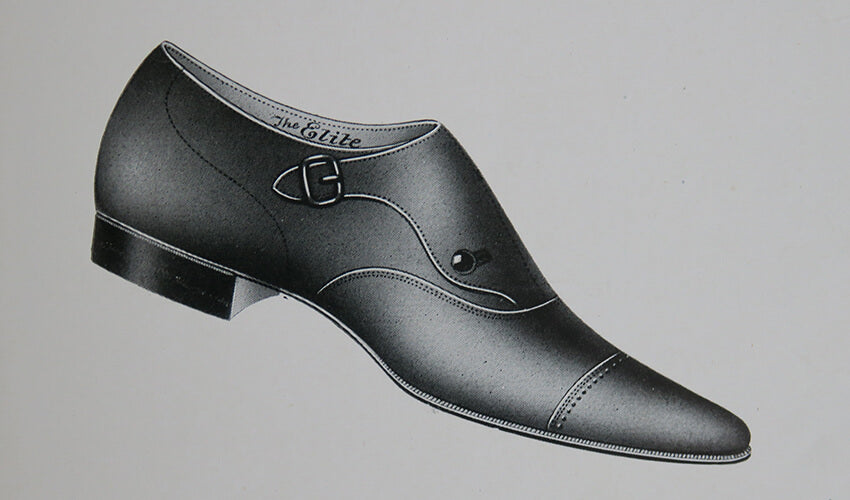This is a detailed illustration of an old-fashioned men's dress shoe set against a light gray to gray-black gradient background. The shoe, shaded in black, features intricate stitching with a pointy toe and a slightly elevated, low heel, approximately an inch thick. The sole is notably thin, emphasizing the classic design. The shoe includes a strap that folds across the top of the foot, securing with a rectangular buckle and a button near the top left. Another prominent detail is the horizontal line across the toe and a wavy stitching line towards the middle. Inside the shoe, the lining, which is lighter in shade, shows cursive text that reads "The Elite." The overall color scheme of the illustration is restricted to shades of black and gray, giving it a minimalist and timeless feel, suitable for a fashion-focused context.